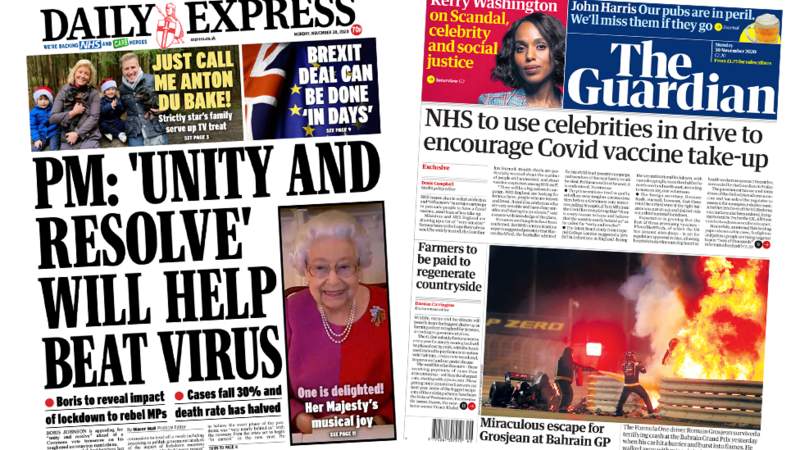The image displays two newspapers side by side, providing a juxtaposition of distinct headlines and themes.

On the left, the newspaper titled "Daily Express" features a collection of various headlines. The upper-left section showcases a heartwarming family image of a husband, wife, little boy, and little girl adorned in Santa Claus hats. Adjacent to this, a British flag headline declares, "Brexit deal can be done in days." Dominating the page is a bold headline emphasizing, "PM: Unity and resolve will help beat virus." In the right section, there is a portrait of Queen Elizabeth accompanied by the caption, "One is delighted: Her Majesty's Musical Joy."

The newspaper on the right, labeled "The Guardian," presents a blend of cultural and topical stories. In the upper-left corner, an article titled "Kerry Washington on Scandal, Celebrity, and Social Justice" features a photograph of the renowned African American actress. Centrally placed, a significant headline reads, "NHS to use celebrities in drive to encourage COVID vaccine take-up," followed by five horizontally aligned paragraphs of text. Toward the bottom right, there is a striking image of two firefighters combating a blaze, with an adjacent article headline, "Farmers to be paid to regenerate countryside." Beneath the image of the fire, another headline notes, "Miraculous escape from Grosjean at Bahrain GP."

Each newspaper presents a snapshot of contemporary issues, distinguished by their unique headlines and accompanying imagery.